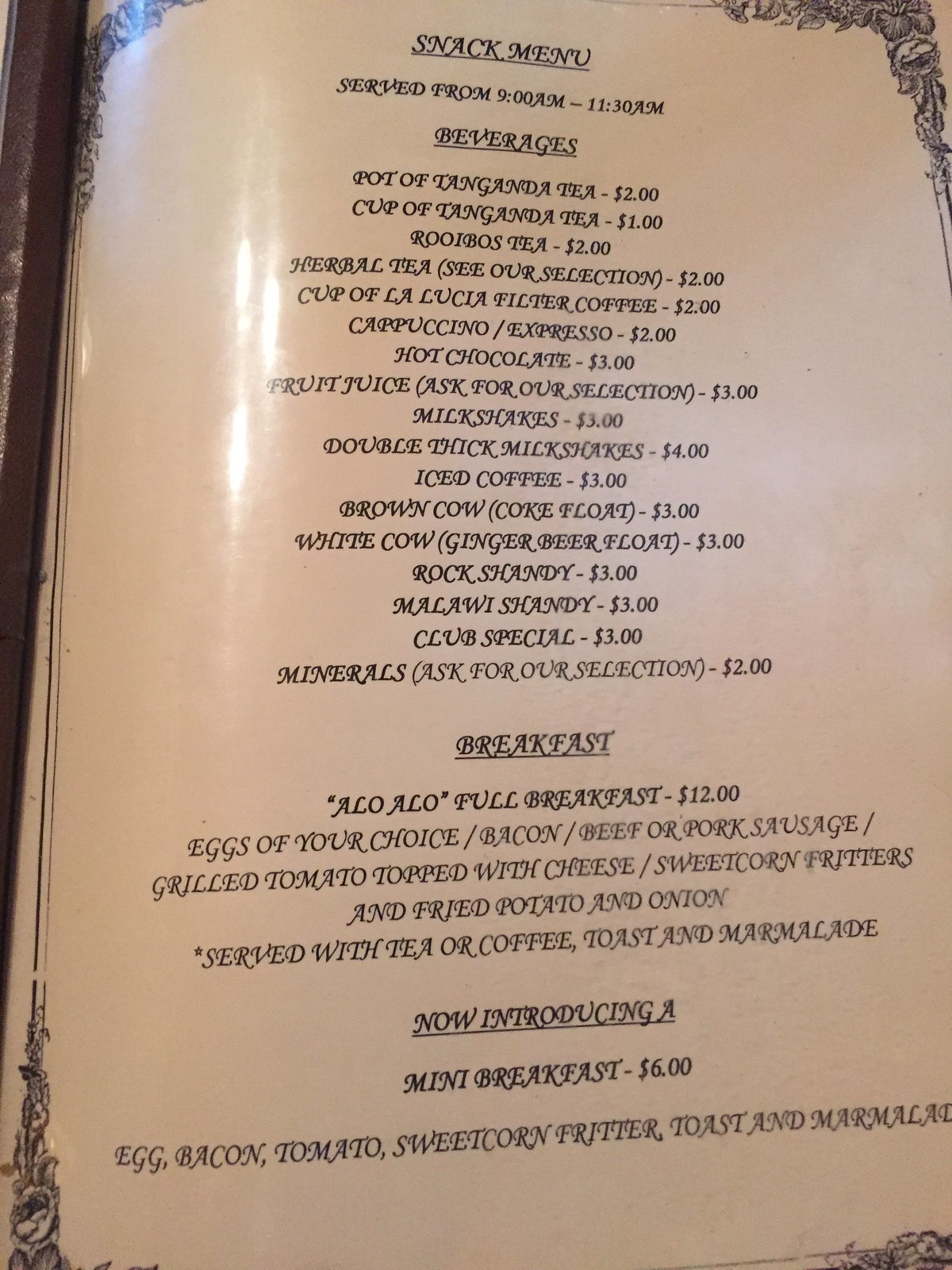The image shows a multi-page menu, primarily focused on breakfast options. The specific page visible is labeled "Snack Menu," indicating that the items listed are available from 9:00 AM to 11:30 AM. The menu features various beverages and breakfast dishes.

One highlighted offering is a "Mini Breakfast" priced at $6, which includes an egg, bacon, tomato, sweet corn fritter, toast, and marmalade. In the beverages section, options include Tanganda tea, herbal tea, hot chocolate for $3, and iced coffee also for $3.

Another notable item is the "Aloe Full Breakfast" priced at $12. This extensive meal includes an egg of your choice, bacon, beef or pork sausage, grilled tomato topped with cheese, and is served with tea or coffee, toast, and marmalade.